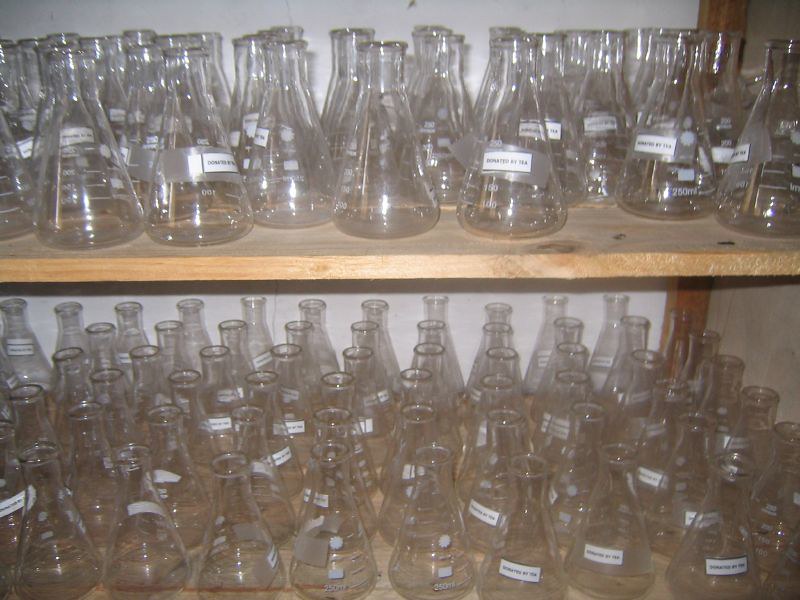This detailed color photograph, taken indoors, showcases two wooden shelves mounted against a stark white wall. The shelves appear to be crafted from yellow pine wood. Each shelf is lined with an extensive array of identical, clear glass beakers, each with a capacity of 250 milliliters. The top shelf contains nearly two dozen beakers, while the bottom shelf holds around three dozen, totaling close to a hundred in the entire image. Each beaker features small measurement markings along its side and is adorned with a small white tag, though the text on the tags is too small and blurry to discern. The beakers resemble scientific flasks or measuring cups, contributing to an organized, laboratory-like appearance.